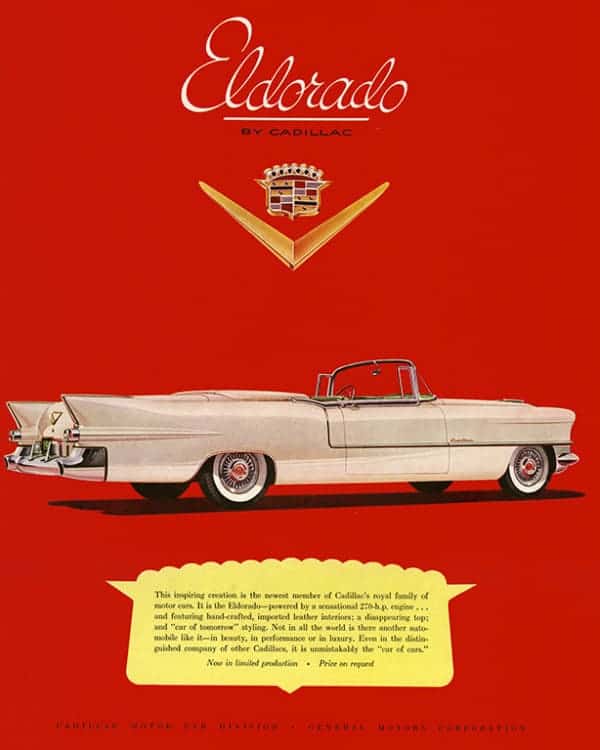This vintage advertisement for the Cadillac Eldorado features a distinctly 1950s aesthetic with its vibrant red backdrop. At the top, in a sophisticated cursive font, "Eldorado" is prominently displayed, underscored by the phrase "by Cadillac" in a refined black font. Below, the iconic Cadillac logo with its regal crest and gold V-shape symbol is prominently showcased. The centerpiece of the ad is a detailed side view illustration of the Eldorado, a classic convertible with its top down, finished in a stylish white with elegant white trim near the bottom and signature Cadillac hubcaps. The illustration is meticulously crafted, evoking the luxurious and low-to-the-ground profile of the era's automotive design. The car is positioned to the right, and while the focus is on the sleek side profile, the trunk and logo are also subtly visible. At the bottom of the advertisement, a yellow square segment contains fine print that presumably elaborates on the car’s features and specifications, though the text is too small and blurred to decipher. This captivating image likely graced the pages of mid-20th-century magazines, enticing readers with its promise of Cadillac elegance and sophistication.